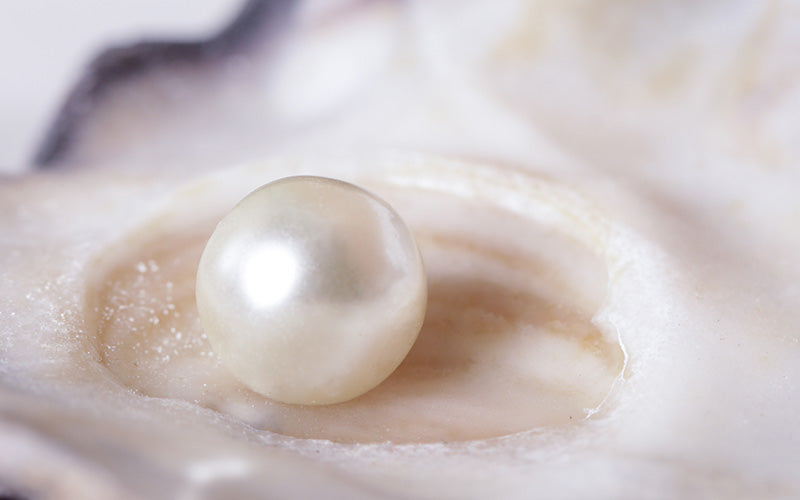This image is a captivating, close-up photograph of a lustrous white pearl nestled within an oyster's interior. The pearl, with its beautiful iridescent shine and silky white color, lies in a central crater-like indentation, surrounded by the oyster's moist, jelly-like flesh. Light refracts off the pearl, adding a glistening effect, particularly noticeable at the top left. The smooth, silky texture of the oyster's interior, contrasted by the darker, purple-black waviness of the shell's border, is clearly visible. Tiny grains of sand also dot the crater to the left of the pearl, further emphasizing the detailed, natural habitat in which the pearl developed. Blurriness in the background provides depth, highlighting the intimate view and the intricate details within the image.